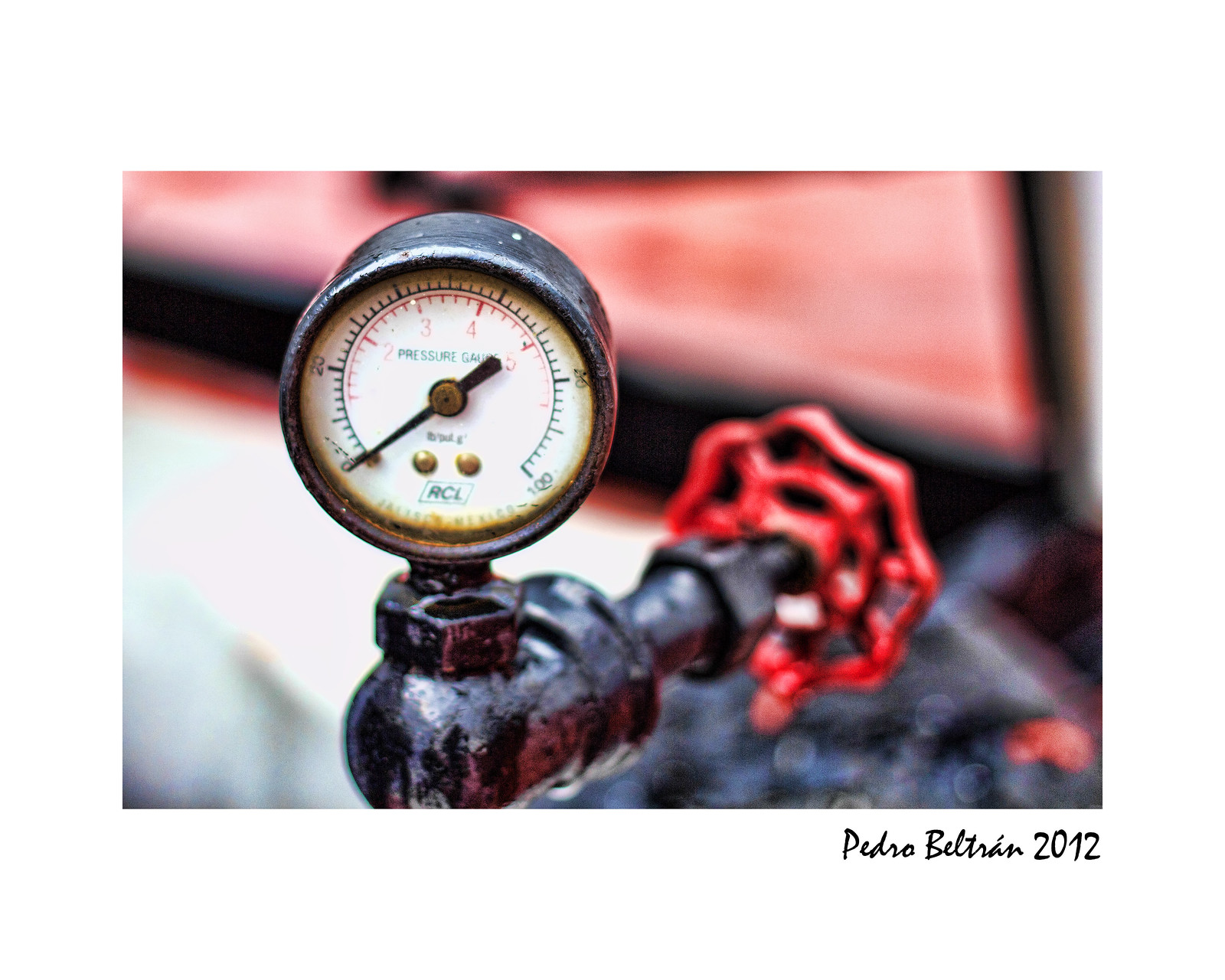The image is a close-up of an old, industrial pressure gauge affixed to a metal pipe with a red, twistable spigot valve situated to the right and slightly behind the gauge. The gauge itself features a white face with green and red sections, marked with numbers from 0 to 100, and includes a central needle, currently pointing to 0. Below the needle, there is a circular section marked with additional numbers ranging from 2 to 5, adorned with notches. The entire assembly has a silver, metallic appearance, conveying a rugged, utilitarian aesthetic. The background is heavily blurred, hinting at some red, white, and gray colors, ensuring all attention is focused on the gauge. In the lower right-hand corner of the image, the name "Pedro Beltran 2012" is distinctly visible, adding a personal and temporal context to the photograph.